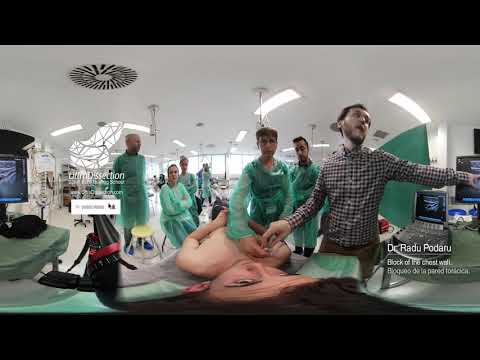This color photograph, presented in a landscape orientation, appears to be a composite of three images documenting a medical training seminar. In the central image, Dr. Radu Padano, dressed in a checkered shirt and sporting a brown beard, is demonstrating a chest wall block technique on a patient who is lying on a bed or stretcher. The patient, likely male, has dark hair flowing towards the camera and is wearing a tan t-shirt. Dr. Padano's hand is shown reaching toward the patient's chest.

Surrounding Dr. Padano, several medical students or emergency technicians, dressed in green surgical gowns, attentively observe the procedure. This scene suggests a non-invasive educational demonstration taking place in a well-lit hospital room, characterized by a white ceiling with a circular vent, various medical instruments scattered throughout, and computer screens positioned on either side of the main activity. In the background, there is a large window.

Distinct from the more central depiction, the left side of the image captures two individuals in surgical scrubs with a monitor and a superimposed graphic, while the right side focuses on Dr. Padano alongside an open laptop with a green screen and other medical equipment. The black horizontal strips at the top and bottom of the photo frame additional details, with the text at the bottom right reading, "Dr. Radu Podaru. Block of the chest wall," followed by unreadable text due to blurring. The image utilizes a fisheye lens effect, adding a distorted, panoramic feel to the hospital scene. The dominant colors in the photo include mint green, white, gray, black, red, purple, tan, and blue.